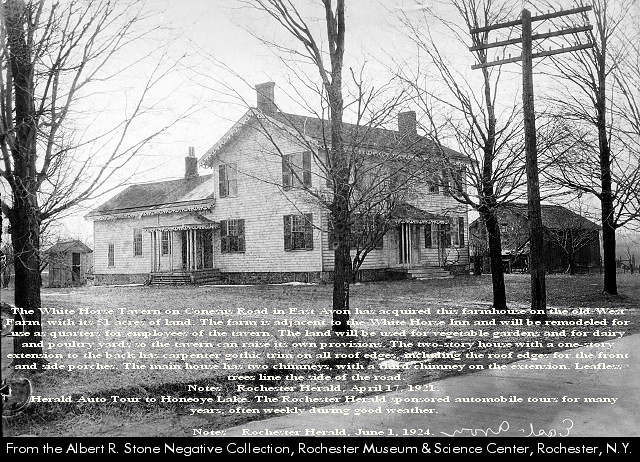The large, square black and white image captures a historic scene with a cloudy sky at the top, revealing a gray and white atmosphere. In the middle, there are several bare trees scattered along the landscape, intersected by a power pole. The focal point is a substantial white wooden farmhouse adorned with many windows and three chimneys visible on its roof. This structure has two covered porch areas, one on the side and one in the front, both with small canopies. A smaller shed is situated behind the house, while a sidewalk and lawn stretch out in front. Bare trees dot the terrain, accentuating the wintery mood.

At the bottom, a partially blurred paragraph of white text provides historical context, mentioning that the White House Tavern on East Avenue has acquired the farmhouse on the Old West Farm. The text implies it was meant to be remodeled for use as quarters for employees, alongside its land being utilized for vegetable gardens, dairy, and poultry provisions for the tavern. At the image's very bottom, a black border contains white text that reads, "From the Albert R. Stone Negative Collection, Rochester Museum and Science Center, Rochester, New York."